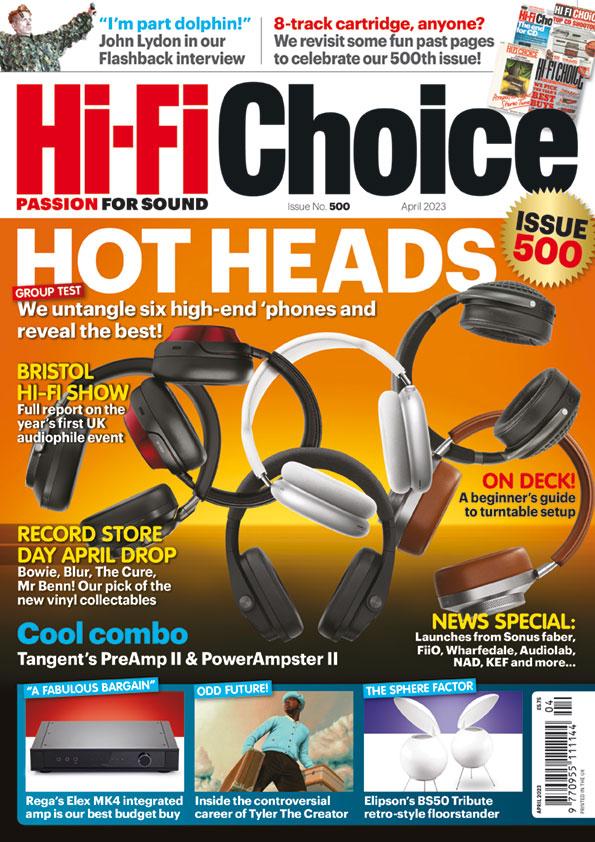This magazine cover features Hi-Fi Choice, celebrating their 500th issue with vibrant red and black lettering headlining "Passion for Sound." The top left announces an exclusive flashback interview with John Lydon under the playful text, "I'm part dolphin." Another top highlight invites readers to revisit memorable moments with "HRack Cartridge anyone," marking the anniversary.

Dominating the cover, an orange and yellow gradient backdrop evokes a sunset, setting the stage for "Hot Heads," a group test of six high-end over-the-head headphones, interlocked, claiming to reveal the best. Complementing this, a gold metallic icon commemorates the milestone issue.

Notable features include the "Bristol Hi-Fi Show," an in-depth report on the UK's premier hi-fi event, and "Record Store Day April Drop," spotlighting new vinyl from Bowie, Blur, The Cure, and Mr. Ben. On the right, "On Deck" offers a beginner’s guide to turntable setup alongside previews of new launches from Sonus Faber, Fiio, Wharfedale, Audiolab, NAD, Kef, and more.

At the bottom, framed by a blue section, the magazine promotes "Cool Combo Tangents Pre-Amp 2 and Power Ampster 2," labeled as a fabulous bargain. Additional articles include "A Fabulous Bargain," featuring the Rekus Alex MK4 integrated amp as the best budget buy, "Odd Future," delving into Tyler the Creator’s career, and "The Sphere Factor," showcasing Ellipson's retro-style BS50 Tribute Floor Stander. Also visible is a barcode located at the bottom right.

Strategically placed subtexts further embellish the cover, promising engaging reads on various hi-fi and cultural topics, neatly tied together to mark this special edition.